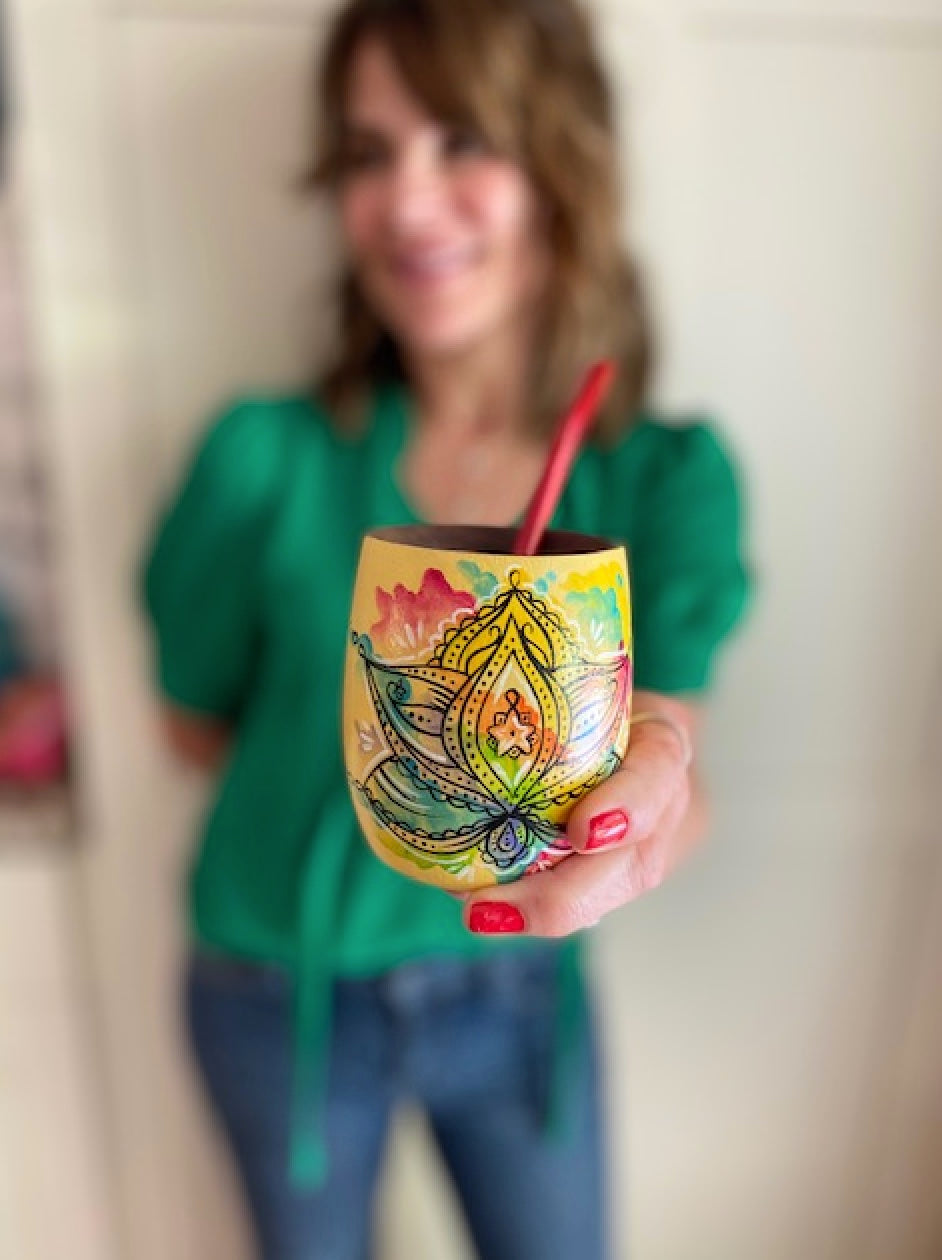This image captures a light-skinned woman with shoulder-length brown hair, standing against an off-white, beige background. She is wearing an emerald green shirt with elbow-length sleeves and dark blue jeans. The woman is blurry and out of focus, making it hard to determine her exact age, which appears to be between 25 to 45 years old. Her face is somewhat visible, showcasing pinkish lipstick. Her right arm is behind her back while her left hand is prominently holding a yellow, opaque cup. The cup, which resembles a stemless wine glass, stands out in clear focus at the center of the image. Adorned with a colorful and intricate design featuring a star and petals in shades of blue, red, green, pink, and orange outlined in black, the cup also has a red bendy straw protruding from it. Two of the woman's fingers holding the cup are clearly visible, showing red-painted nails and a ring on her index finger. The interior of the cup appears to be brown. This composition creates a striking contrast between the blurred background and the vividly detailed cup in the foreground.